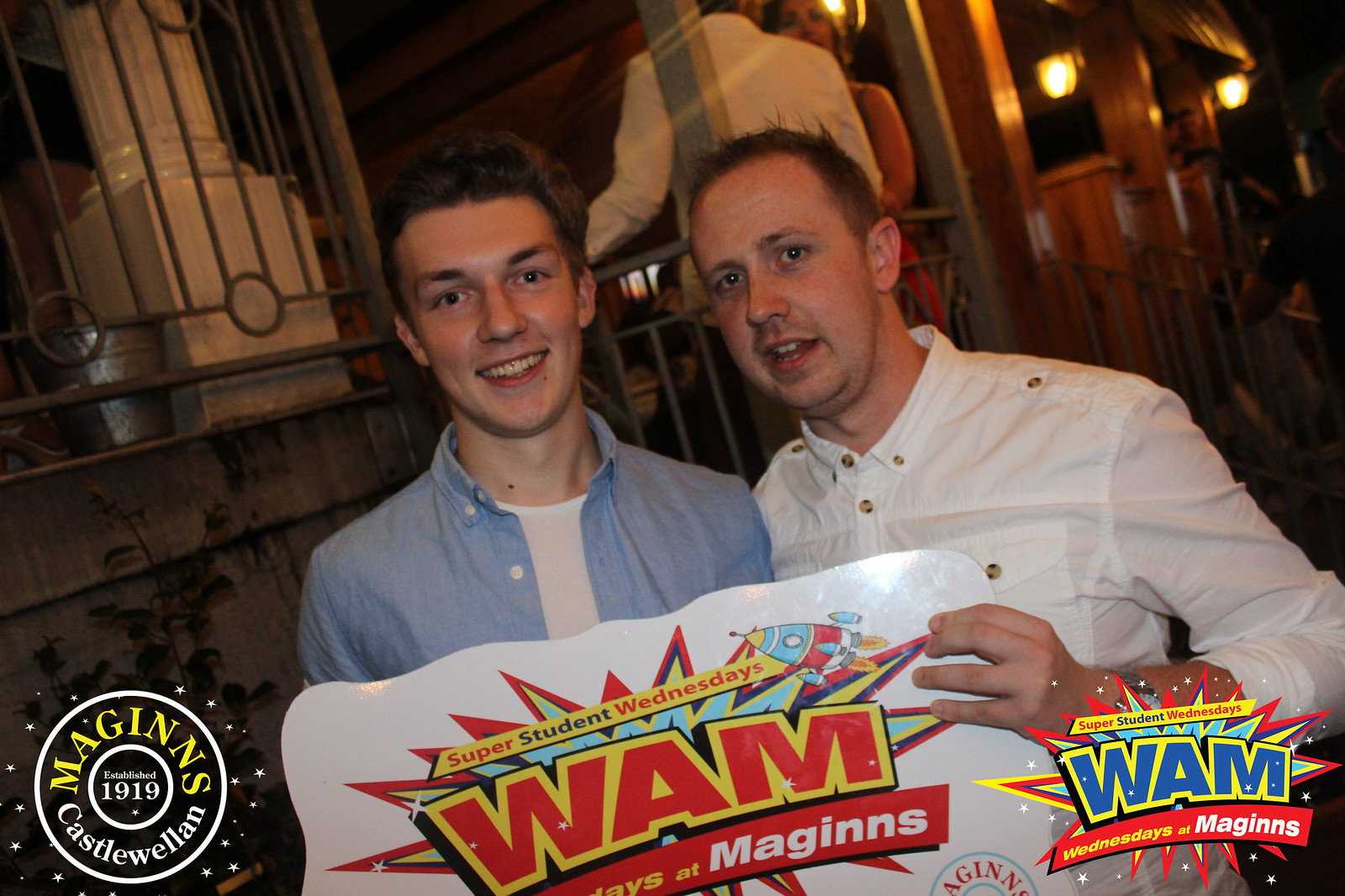This image, rectangular in shape and likely taken outdoors at night under artificial lighting, captures a scene with a backdrop of a sky that's pitch black, suggesting a nighttime setting. The photograph features a patio area raised behind two gentlemen standing at the center. The patio is enclosed with an iron railing, and a staircase with a matching railing ascends to it on the right side of the image. The patio structure includes wooden beams and white-painted columns, adding a touch of architectural elegance.

The focal point of the image is the two gentlemen posing for the camera. The man on the left has dark hair and is dressed in a blue collared shirt with a white t-shirt underneath. His companion on the right also sports dark short hair and is attired in a white collared shirt. Both men are holding up a sign that reads, "Super Student Wednesdays Wham at McGinn's."

Imposed in the lower left corner of the photograph is a logo for McGinn's, detailing "Established 1919, Castle Welland." In the lower right corner, another logo reiterates the promotion, "Super Student Wednesdays Wham," along with "Wednesdays at McGinn's." This detailed composition indicates a promotional photograph taken to highlight an event or offer at McGinn's pub or restaurant.